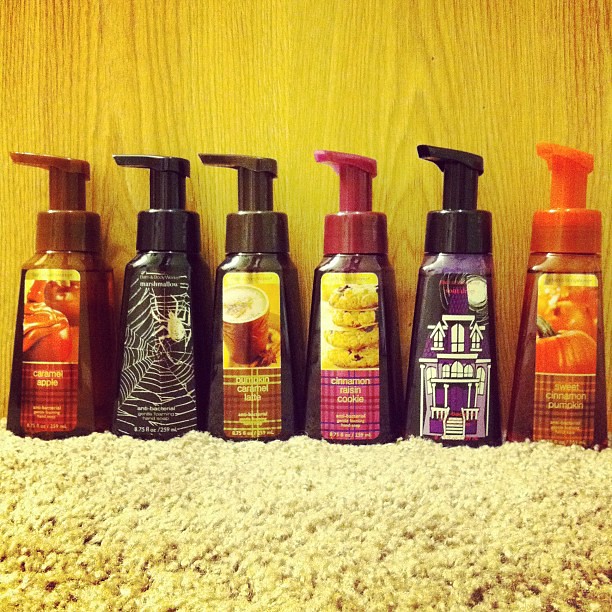The image is a color photograph featuring a lineup of six plastic pump bottles, likely for foaming hand soap, arranged horizontally on a fuzzy, oatmeal-colored shag carpet or bath mat. The backdrop is a wooden surface with a vertical grain pattern. The overall tone of the photo has a slightly yellowish filter. The bottles are rectangular and identical in shape, standing about 10 inches tall, with their pump spouts facing three-quarters to the left.

The labels on the bottles are autumn-themed with various colors and designs. From left to right, the details on the bottles are as follows:

1. The first bottle has a brown pump top and features an image of apples with text that includes the word “apple.”
2. The second bottle includes Halloween imagery with a spider and spiderweb, and has a black pump top.
3. The third bottle, also with a brown pump top, has a label indicating "cinnamon caramel latte."
4. The fourth bottle, featuring a purple pump top, reads "cinnamon raisin cookie."
5. The fifth bottle has a Halloween-themed label with a haunted house in purple and white and a black pump top.
6. The final bottle sports an orange pump top and says "sweet cinnamon pumpkin."

These bottles are reminiscent of those found at stores like Bed Bath & Beyond or Bath and Body Shop, featuring various autumn and Halloween scents.